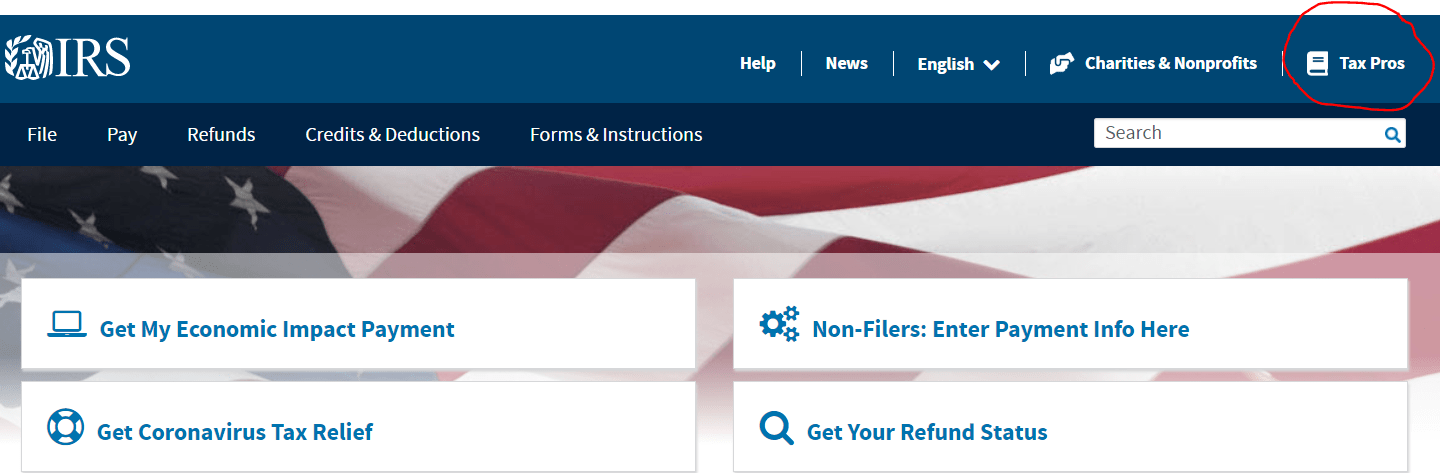The image displays the top section of the IRS website. The upper left corner prominently features "IRS," while a dark blue banner spans the top of the page, displaying white-text links including "Help," "News," "English" (with a dropdown for language selection), "Charities & Nonprofits," and "Tax Pro." The "Tax Pro" link is emphasized with a red circle. Beneath this, a second, navy blue bar offers additional links: "File," "Pay," "Refunds," "Credits & Deductions," "Forms & Instructions," and a search box on the far right. The background showcases an American flag. Positioned below this are four clickable boxes labeled "Get My Economic Impact Payment," "Get Coronavirus Tax Relief," "Non-Filers: Enter Payment Info Here," and "Get Your Refund Status."